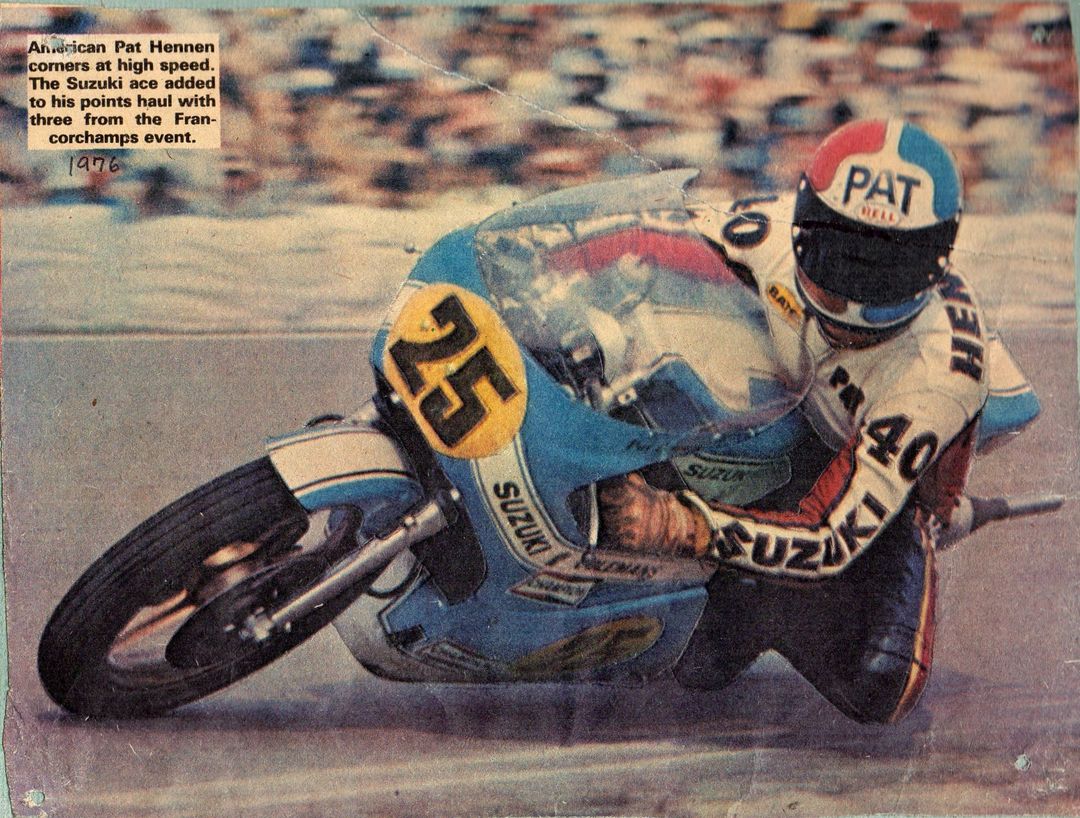The image is an action-packed color photograph from 1976, capturing American motorcycle racer Pat Hennon taking a sharp turn at high speed during a race. Despite the photo's poor quality, marked by scratches, watermarks, and dust, the dynamic moment shines through. Pat Hennon is donning black leather pants and a striking white and red jacket emblazoned with "Suzuki" and the number 40 in black lettering. His red, white, and blue helmet displays the name "PAT" across the top with a dark black visor. Hennon's blue motorcycle, featuring a yellow circle with the black number 25, is the focal point as it leans into the turn to the left side of the frame. Blurred spectators in the background highlight the intense speed of this moment. The top-left corner of the image includes the printed caption, "American Pat Hennon corners at high speed. The Suzuki ace added to his points haul with three from the Franco Champs event, 1976," providing context and historical significance to this thrilling depiction.